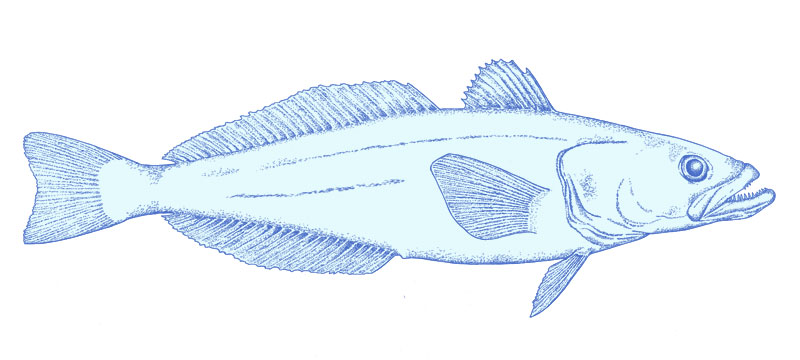This is an intricately hand-drawn image of a long, narrow fish against a plain white background. The fish is oriented horizontally with its tail on the left and its head on the right, as if swimming towards the right. Rendered in dark blue for the outline and filled with a lighter blue for its body, the illustration aims for a realistic yet artistic effect, resembling a detailed pencil or art pen sketch. The head of the fish features a slightly open mouth revealing sharp teeth and a black eye that gazes slightly upwards to the right. The fish's body showcases delicate striping details, with one stripe running near the top of the body and another just below it, stopping before the side fin. The fins are meticulously placed, including a small one below the gills, a side fin, a short dorsal fin on top, a longer dorsal fin along the back, and another fin running along the bottom near the tail. The overall color scheme and detailed anatomical features evoke a sense of realism combined with the clear hand-drawn quality.